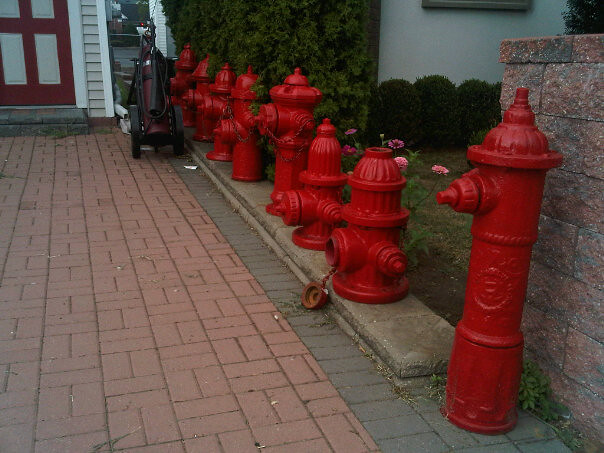In this outdoor evening scene, a row of eight red fire hydrants, each differing in design and height, lines a curb adjacent to a lower retaining wall. The tallest hydrant, positioned off the curb, stands against a chest-high, light pink brick wall, situated in front of a shorter brick wall. Beyond the hydrants lies a field adorned with pink flowers and lush green grass. To the left, the walkway features a driveway bordered by gray and reddish-brown bricks. A red door with four white rectangular strips is visible on a white-walled home or shed. Additionally, a piece of equipment resembling a golf bag on wheels with a vacuum attachment is spotted in the vicinity, contributing to the eclectic arrangement.